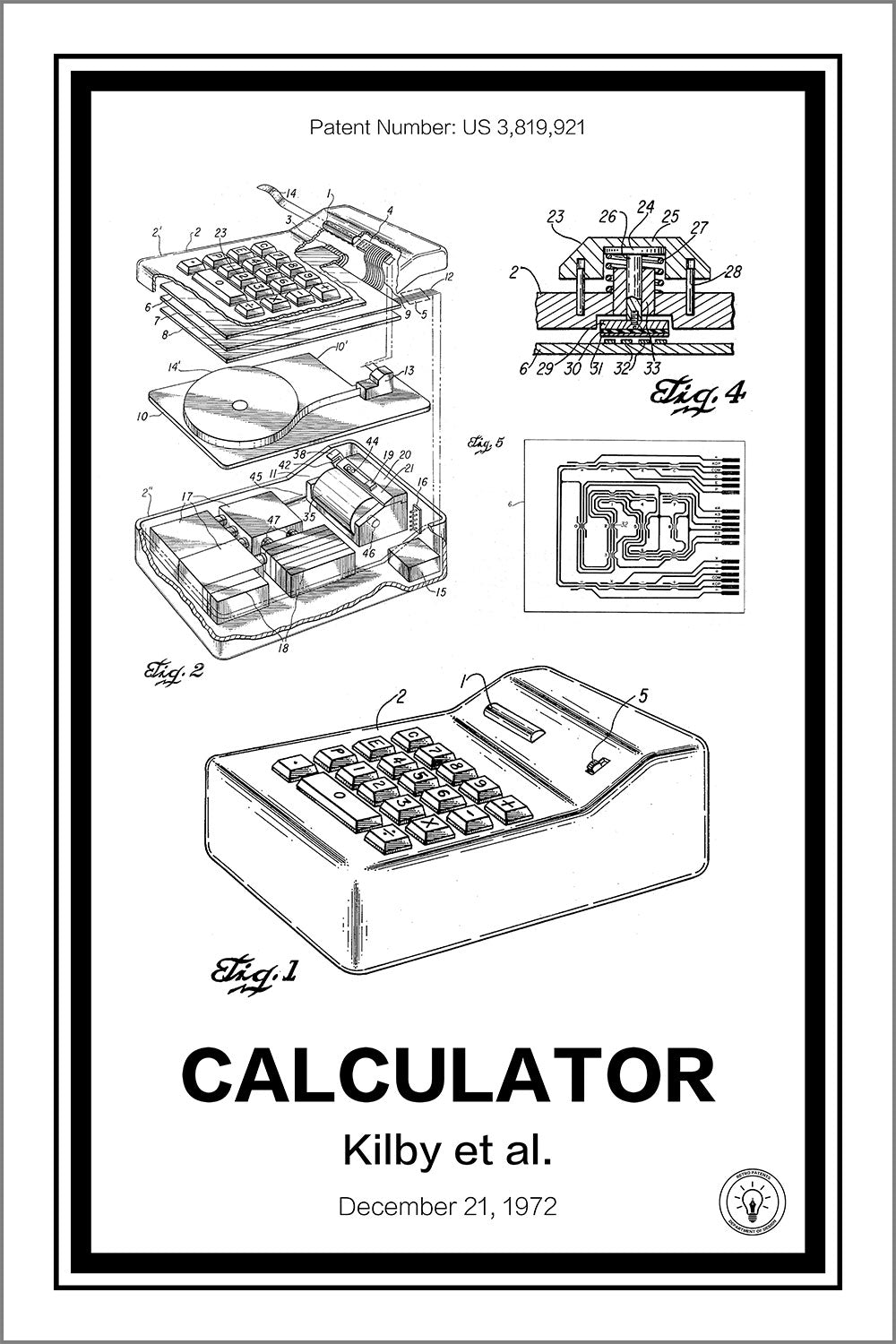This detailed poster illustration of a calculator displays a comprehensive breakdown of its design and inner workings, featuring patent number U.S. 3,819,921 prominently at the top in black text. At the bottom, "Calculator, Kilby et al, December 21st, 1972" is clearly inscribed. The poster includes five distinct images of the calculator: the top left section portrays the device in various stages of disassembly, revealing internal components; another image shows a detailed view of the internal computer chip; another depicts the calculator partially assembled with its top lifted; and a full, assembled view of the calculator is presented below, as it would appear ready for use. The illustrations, borders, and text are all rendered in black ink on a white background, with three concentric black borders framing the entire poster. Additionally, a logo featuring a circle with a stylized light bulb is positioned at the bottom right corner.